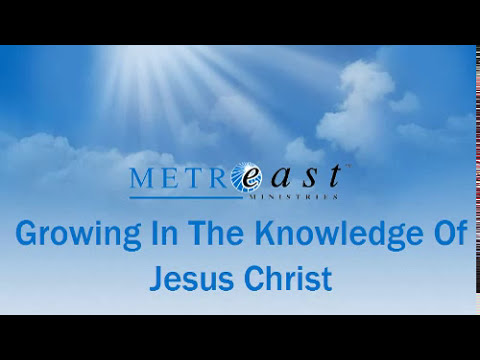The image serves as a promotional piece for Metro East Ministries. The background portrays a serene blue sky adorned with wispy white clouds. In the upper left corner, beams of sunlight pierce through the sky, creating a radiant effect though the sun itself is not visible. The centerpiece of the image features the text "METRO EAST MINISTRIES," with the “E” artistically integrated into the “O” of "METRO" to form a globe design. Below this, in larger blue letters, the text reads, “GROWING IN THE KNOWLEDGE OF JESUS CHRIST.” The image is framed by two thick horizontal black bars, one at the top and one at the bottom, adding a polished border to the design. Additionally, a thin sliver of red, black, and white can be seen along the right edge of the image.